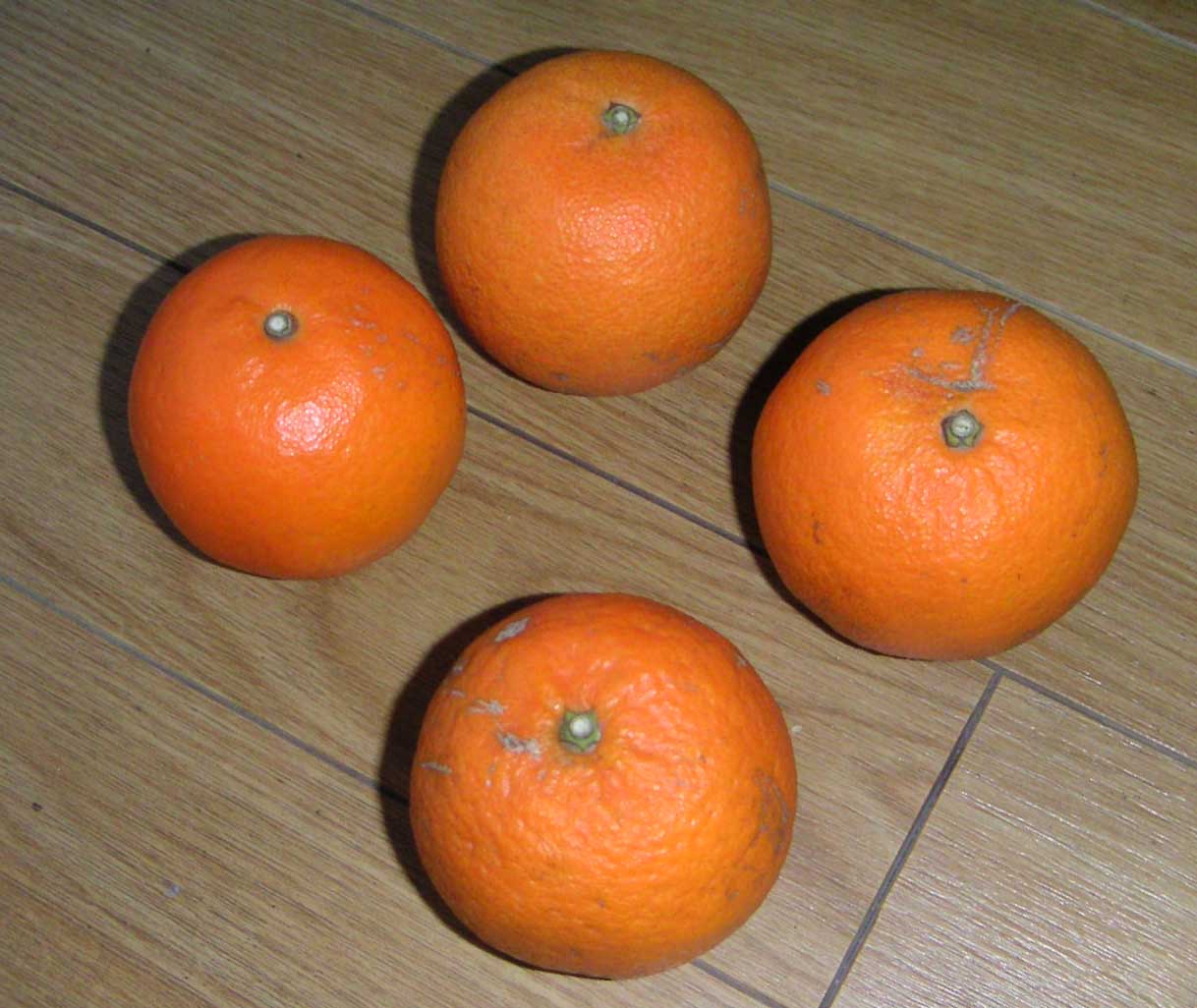This top-down photograph, taken with a flash and set against a light brown hardwood floor with cement linings, shows four unpeeled oranges arranged in a diamond shape. The light source comes from the bottom right, emphasizing the vibrant orange skin of the fruits. However, the oranges exhibit varying degrees of aging and imperfection. The orange on the left appears to be the freshest, with the most vivid color and intact skin. Moving clockwise, the top orange shows slight aging with a duller rind, while the right orange has begun to develop some mold, indicating more significant aging. The bottom orange is the most deteriorated, displaying the palest rind and the most mold growth. Imperfections such as browning, rough texture, and cracks are visible on the skins of all the oranges, highlighting their natural wear.